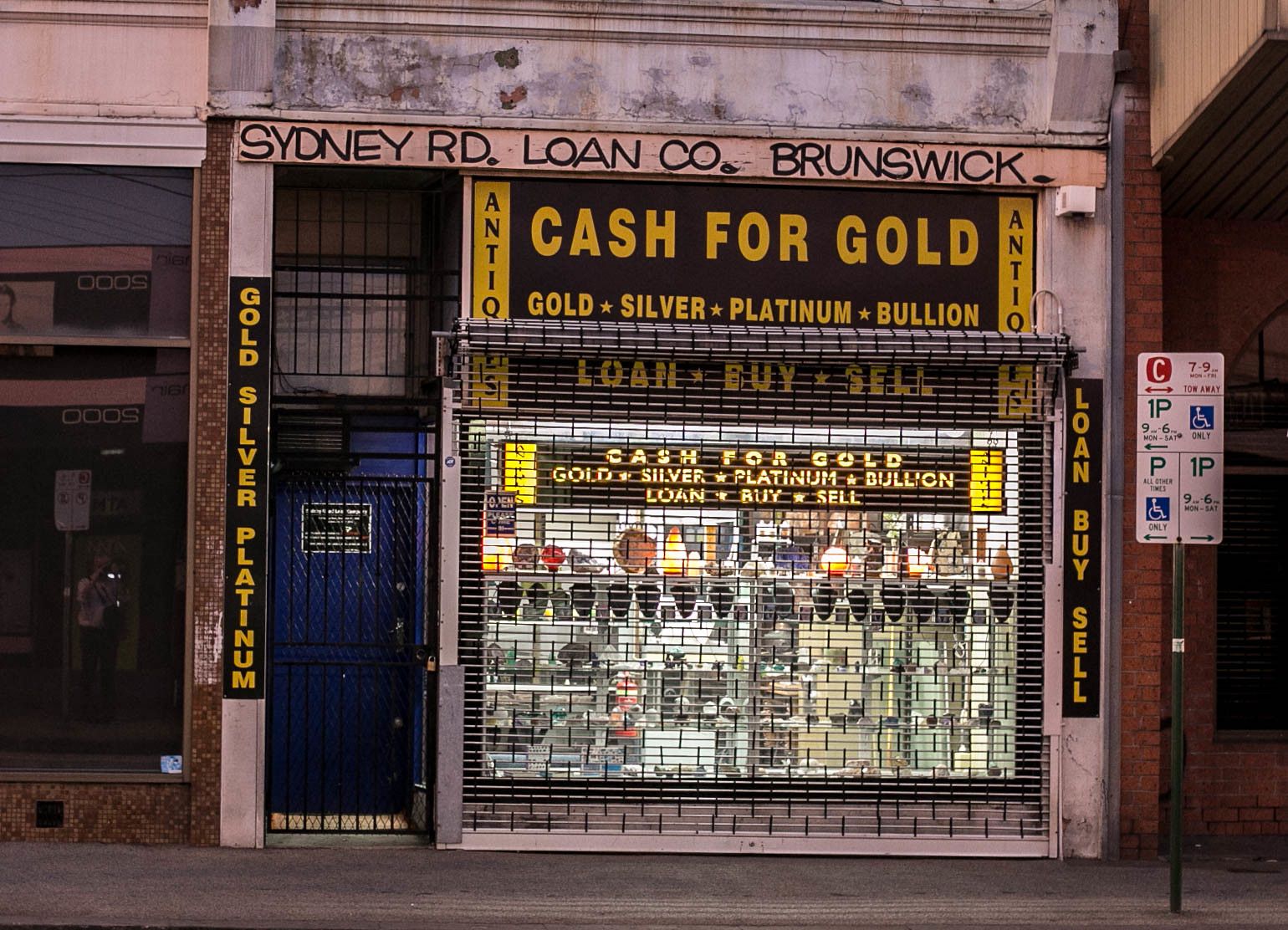This detailed landscape-oriented color photograph depicts the front of a retail shop located on Sydney Road, labeled as Lonscoe, Brunswick. The prominent sign across the top displays "Cash for Gold" in yellow letters against a black background, accompanied by the words "Gold, Silver, Platinum, Bullion, Loan, Buy, Sell." Flanking this central sign, the words "Antiques" are displayed vertically on both sides in black letters on a yellow background. The entrance of the store features a blue door secured by a metal gate to the left side of the window. The window itself is protected by a black mesh security screen, obscuring the items inside. On the left side of the building, a vertical sign reads "Gold, Silver, Platinum," and on the right, a similar vertical sign states "Loan, Buy, Sell." Additionally, on the far right, a parking sign mounted on a pole provides detailed parking regulations and includes a wheelchair accessible symbol. The building façade is framed between adjoining structures with visible brickwork.